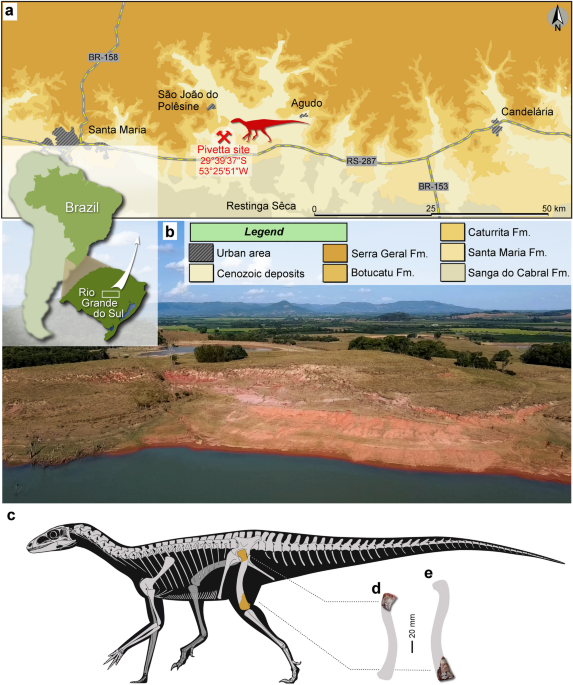The image, resembling a detailed textbook illustration, is vertically oriented and features a series of graphics and photos related to the discovery site of a dinosaur in Brazil. At the top, there's a map in English highlighting South America with Brazil emphasized, pinpointing specific locations like Santa Maria, Candelaria, and the Piveta site with coordinates 29°39′37″S, 53°25′51″W, where the dinosaur was found. Illustration A presents the geographic distribution of the dinosaur, covering areas such as Santa Maria and Sao Jose de Palestina. Following this, Illustration B illustrates a color-coded map legend indicating different urban areas and geological deposits, including Sarazonic Deposits and various Formations like Sara General FM and Santa de Cabrillo. This section also includes an actual photograph of the discovery site characterized by flat red dirt, a pond, and green mountains in the background. Below this, Illustration C depicts a drawn image of the dinosaur's skeletal anatomy with distinguished bone colors, providing a comprehensive view of its structure.